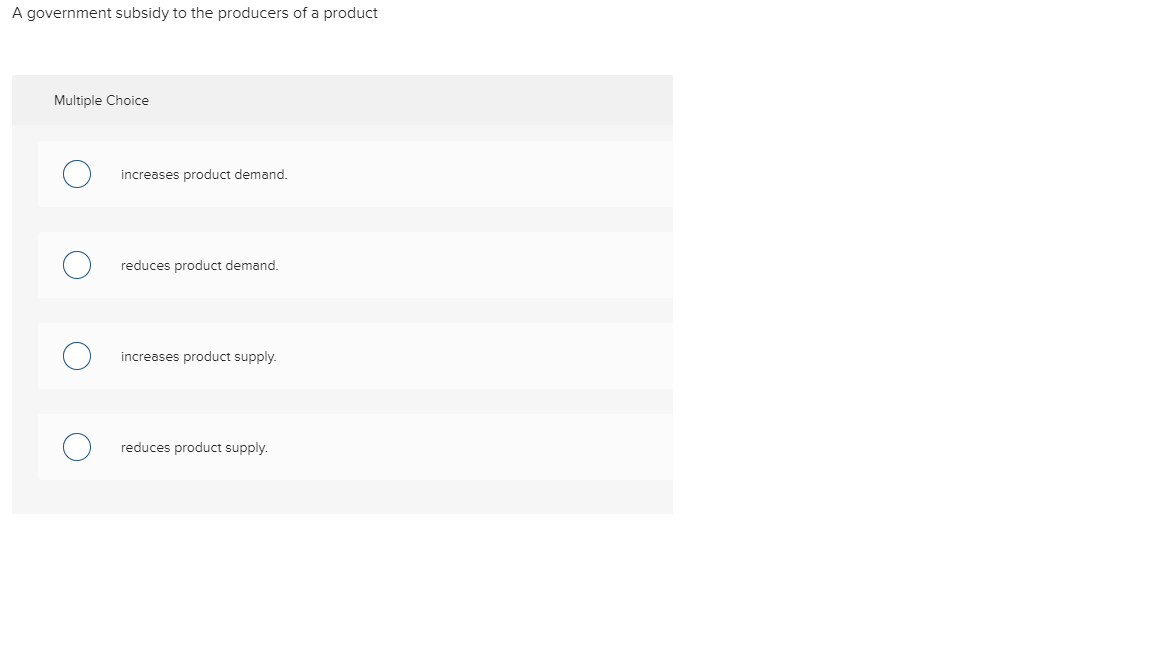The image depicts a section of what appears to be a government-issued multiple-choice test. The background is stark white with very minimalistic design elements. At the top, a question is presented in small, plain text: "The government subsidy to the producer of a product." Below this question is a light gray box labeled "Multiple Choice," containing four potential answers, each within its own slightly lighter gray or white sub-box.

The answers listed are:
1. Increases product demand
2. Reduces product demand
3. Increases product supply
4. Reduces product supply

Each option is accompanied by a clickable bubble on its left, though none of these bubbles have been filled in, indicating no selection has been made. There is no indication of the question number or additional context, reinforcing the simplistic and understated design of the test. The overall layout implies this image is part of a standardized assessment, potentially used for evaluating economic understanding of government subsidies.